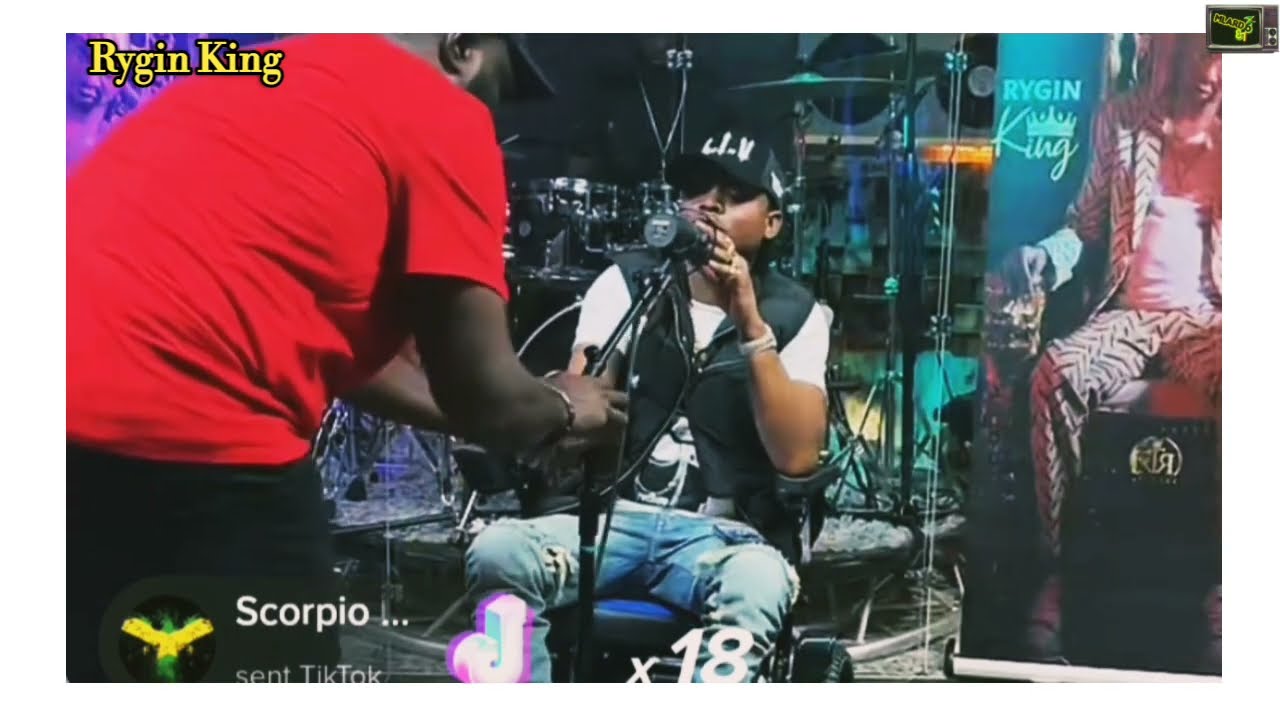In the image, a black man is seated, speaking into a large microphone that casts a shadow across his eyes. He is wearing a black baseball cap that says "L.I.V." in white letters, a black, unzipped vest over a white t-shirt, and ripped blue jeans. His elbows rest on the armrests of his chair. Standing to his left, a large black man in a red t-shirt and black pants is adjusting the microphone. Behind the seated man is a drum set featuring a black drum and a cymbal above his head. In the top left corner of the image, "Raijin King" is written in yellow with a green outline. At the bottom left, "Scorpio" and "Saint Tick Tock" are displayed in white. There is also an icon of a person with yellow arms and green head and legs. Additionally, beneath the man’s knee, the number "18" with an “X” in front of it is visible. On the far right side of the image, a banner with "R-Y-G-I-N King" in blue letters and a crown above the "I-N-G" is present, alongside a picture of a man in a patterned suit sitting on a high chair. Furthermore, a white "J" with a pink outline is also noticeable near the bottom center. The overall scene suggests a live stream setup, possibly for a musical performance.